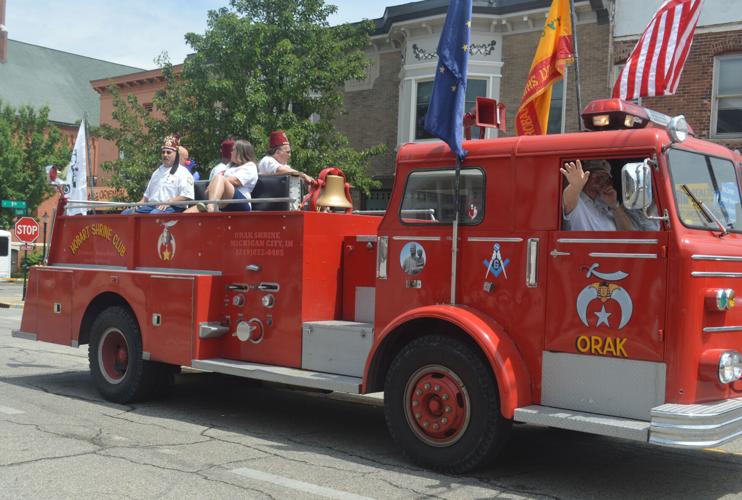An old, likely decommissioned fire truck is driving to the right on a grey road marked with white lines, part of what seems to be a parade. The truck, sponsored by the Shriners Club, bears multiple flags - an American flag, a yellow and red flag, and a blue flag on its roof, along with one more at the back. The front and sides of the truck feature notable symbols including the Shriner emblem with a sword and crescent, alongside the text "ORAK" in capital yellow letters. The driver's side door has additional white and yellow signs, plus another symbol resembling a triangle with a V, encasing a circular portrait, possibly of the owner. 

A man in a white shirt and sunglasses is behind the wheel, his arm out the window, possibly coughing. The back of the truck has been modified with benches for parades, where men and women in white shirts and red fezzes with black tassels sit, facing the sides. Two people are on the near side, and three are on the far side, some looking towards the back. The parade route passes by tall brick buildings, perhaps including a courthouse, with green trees visible in the background and a stop sign at a corner.